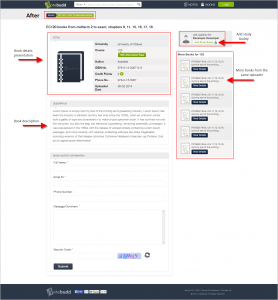The screenshot depicts a cluttered webpage that appears to be either a tutorial or an instructional guide for a website related to customizable products, such as notebooks or books that users can create themselves. Due to the image being minimized or scaled down, the font size is extremely small, rendering the text almost illegible. The page features various design elements, including an image of a notebook or book and numerous clickable options likely intended for customization or listing products for sale.

Key sections of the webpage are highlighted with red outlines and boxes, emphasizing their importance. Red arrows point to different areas, suggesting where to input information or where specific actions should be taken. There is also a segment dedicated to user profiles, possibly indicating that users can sign in or create accounts to manage their listings. Despite the informative layout, the tiny font size makes it challenging to discern the exact instructions or descriptions.